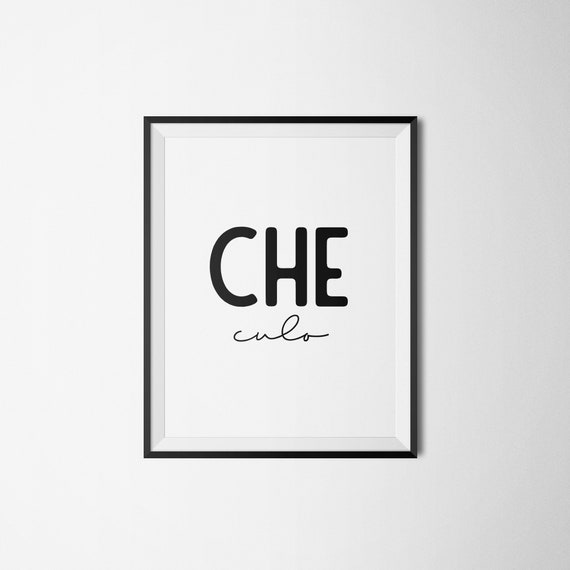The image is a full-color photograph of a vertically rectangular, monochromatic artwork without a border. The backdrop of the overall image is off-white, gradually becoming more washed out towards the bottom-left corner. Central to the image is a black frame containing a piece of paper with a white background. On this paper, three letters, "C," "H," and "E," appear in either dark brown or black uppercase text. Directly below these letters, there are lowercase cursive letters spelling "C-U-L-O." There is a slight shadow cast by the frame onto the off-white background, adding depth to the composition. The artwork does not provide additional context or words beyond the prominent text within the frame, leaving the viewer to interpret its meaning, possibly alluding to the famous revolutionary "Che."